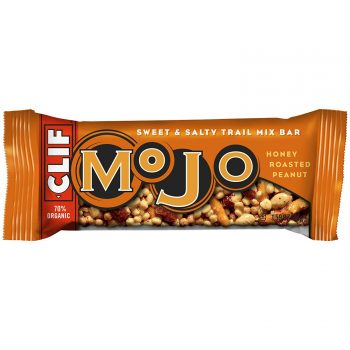This is an image of a single-serving, sweet and salty trail mix bar with prominent branding. The bar has a distinctive yellow wrapper with the centerpiece being the word "MOJO" in large, bold letters. Each letter in "MOJO" is outlined in black and encircled with brown, except for the "J" which features mostly black with a smaller brown outline. Above "MOJO," in a smaller white font, the packaging reads "Sweet and Salty Trail Mix Bar." To the right of "MOJO," it says "Honey Roasted Peanut." The wrapper showcases a small window under the MOJO letters, possibly displaying the actual granola bar or an image of it, complete with a mix of almonds and various grains. 

On the left side, a red vertical panel displays the brand name "CLIF" in all caps white font. Below the brand name, it indicates that the product is either 70 or 79 percent organic. The overall design is horizontal, making it easy to read the information when the bar is placed flat. The packaging’s vibrant colors and strategic placement of text and images emphasize the MOJO brand, the trail mix's flavor, and its organic ingredients.